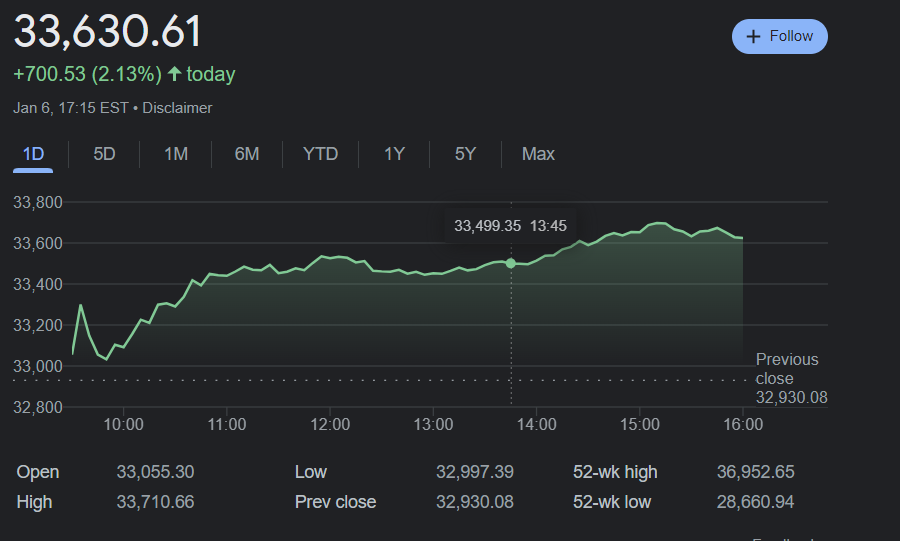A detailed financial display is depicted on a screen with a sleek black background and sharp white or green lettering. The focal point of the image is the striking value of 33,630.61, presumably representing the current value of a stock or index. A secondary figure, showing an increase of $700.53 for the day, is also prominently featured, highlighting the day's positive performance. The display allows users to select various time frames to view the data trend, including options for one day, five days, and a month. Additionally, the lower section of the screen provides a comprehensive breakdown of essential financial metrics: today's opening value, the day's highest and lowest values, the previous closing value, as well as the 52-week high and low points. Notably, there is no specific mention of the company or index related to these financial figures, which might be an intentional omission, possibly for privacy reasons.